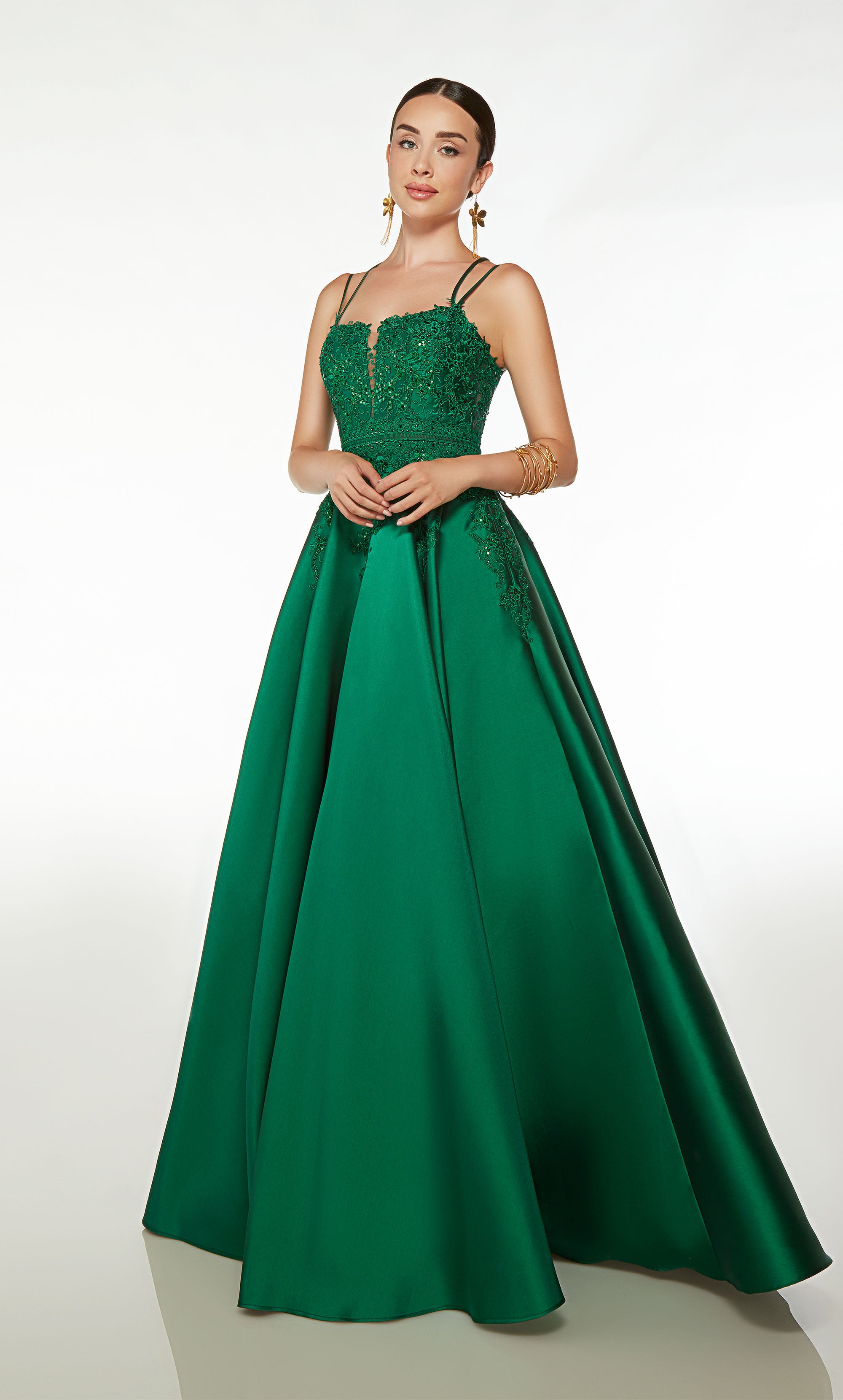This is a photograph of a fair-skinned Latina woman standing tall against a white background with a slight shadow beneath her feet. She is wearing an elegant forest green evening gown that reaches the floor, with thin shoulder straps and a textured, sparkly top that features intricate green, ribbon-like decorations. The rest of the dress flows smoothly downwards. Her pose is composed, with both hands resting in front of her stomach, tilting slightly to her right. She is adorned with gold jewelry, including several gold bracelets on her left forearm and five-petaled gold flower earrings that dangle below her ears. Her straight black hair is parted down the middle and slicked back into a low bun. She has a serious expression, enhanced by her makeup which includes red lipstick.